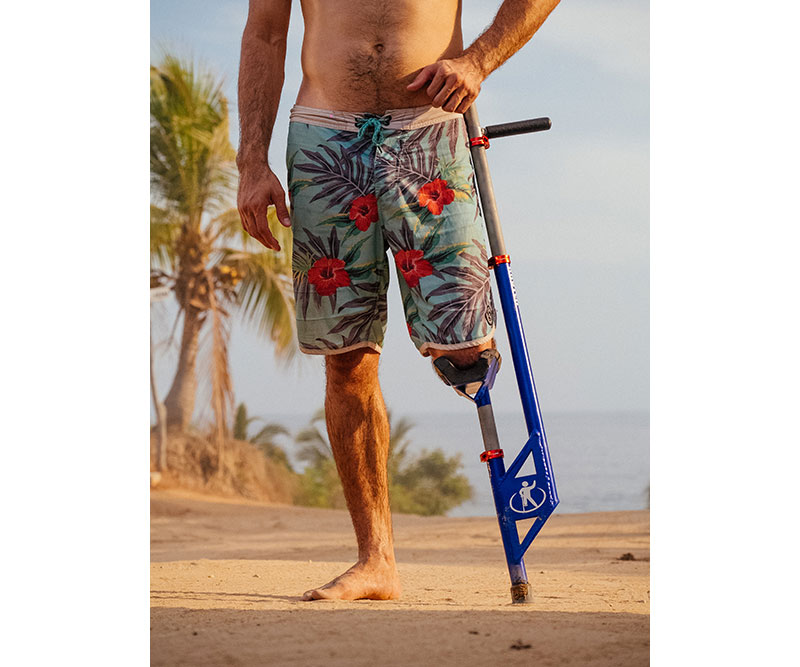The photograph depicts a man standing on a sandy beach with his left leg amputated at the knee. He has light skin with visible body hair on his lower abdomen, forearms, and right leg. He is shirtless and wearing light blue shorts adorned with orange and red tropical flower patterns. His left leg rests on a blue metal crutch-like device designed to support the knee, which features a small black handle that extends up the side of his body. In the background, there is a serene beach setting with sand leading up to the edge of the ocean, palm trees on the left, and a clear blue sky overhead with no significant cloud cover.